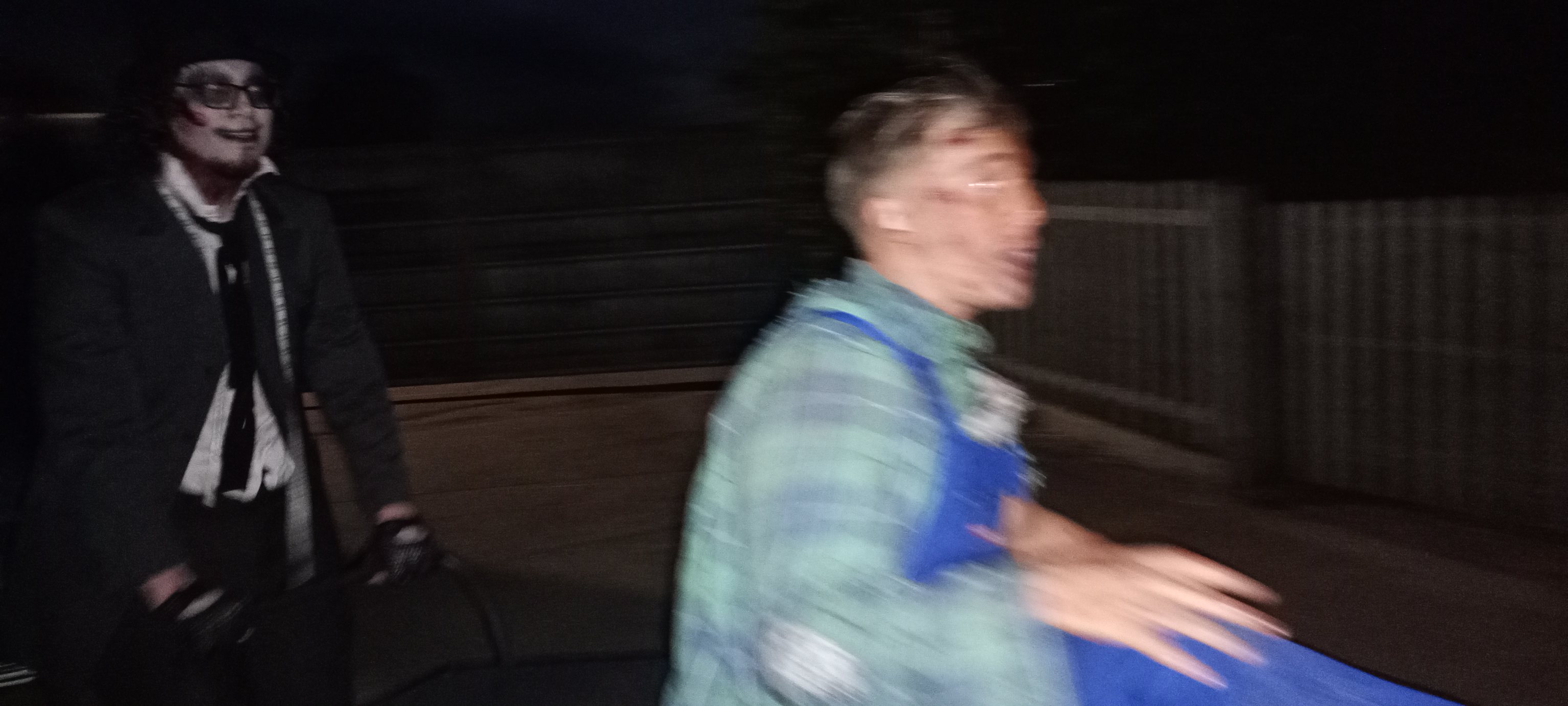Two individuals are dressed in elaborate costumes. The person in the foreground is wearing a green checkered shirt and has a blue accessory on their chest. Their face is smeared with dirt makeup and fake blood, creating a frantic and distressed appearance. They seem to be walking forward with a sense of urgency. Behind them to the right is a white metal fence. Further back, another person is visible in a costume. This second individual has their face painted white, with a red cut and dark shading around their eyes, giving a haunting effect. They are wearing glasses, a suit with a black tie, and black UFC gloves. This person is pushing a shopping cart or stroller. The ground behind both of them is sandy.